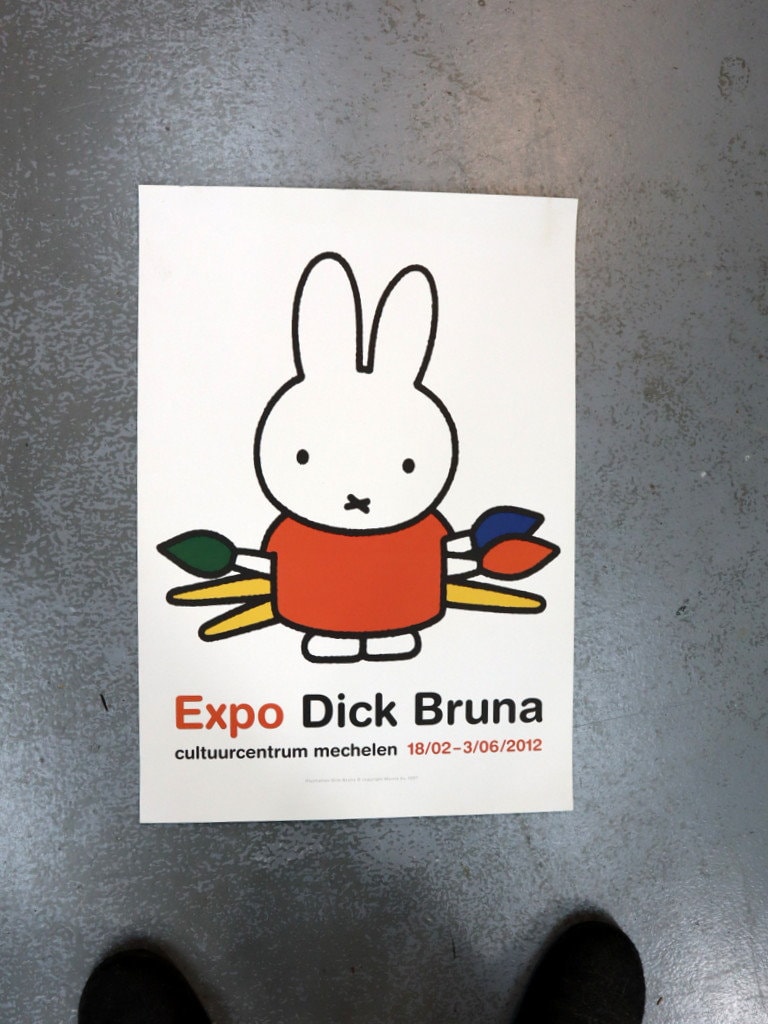The image shows a poster lying flat on a gray floor, with the top parts of two black shoes visible at the bottom, suggesting someone is standing and looking down at it. The poster features a white bunny with black dot eyes and an X for a mouth, wearing a red shirt. The bunny is holding three paintbrushes with wooden handles; the brush tips are colored blue, red, and green. The poster has text beneath the bunny in red and black lettering that reads: "Expo Dick Bruna. Culture Centrum Michelin." There is also a date, 18-02-362012, written in red.